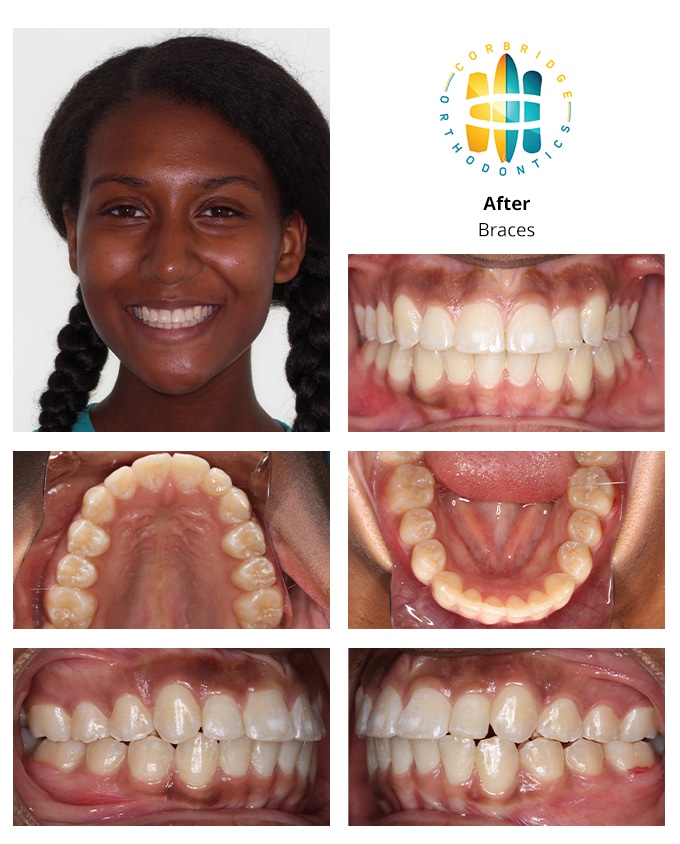The image is a rectangular collage featuring a series of photographs focused on a young woman's dental transformation, with the overall aspect ratio making the longer sides twice the length of the shorter sides. In the top left corner, a close-up shot shows the smiling face of a young Black woman with dark hair styled in two braided ponytails, wearing a blue shirt. The background is solid white. To the right, prominently in the top right corner, is a logo in green and blue that reads "Core Bridge Orthodontics," with black text beneath it stating "After Braces." Below the woman's photo are five close-up images showcasing her teeth from various angles, including a downward view of her upper teeth. These images highlight the results of her orthodontic treatment, providing detailed visual evidence of her straightened, white teeth.